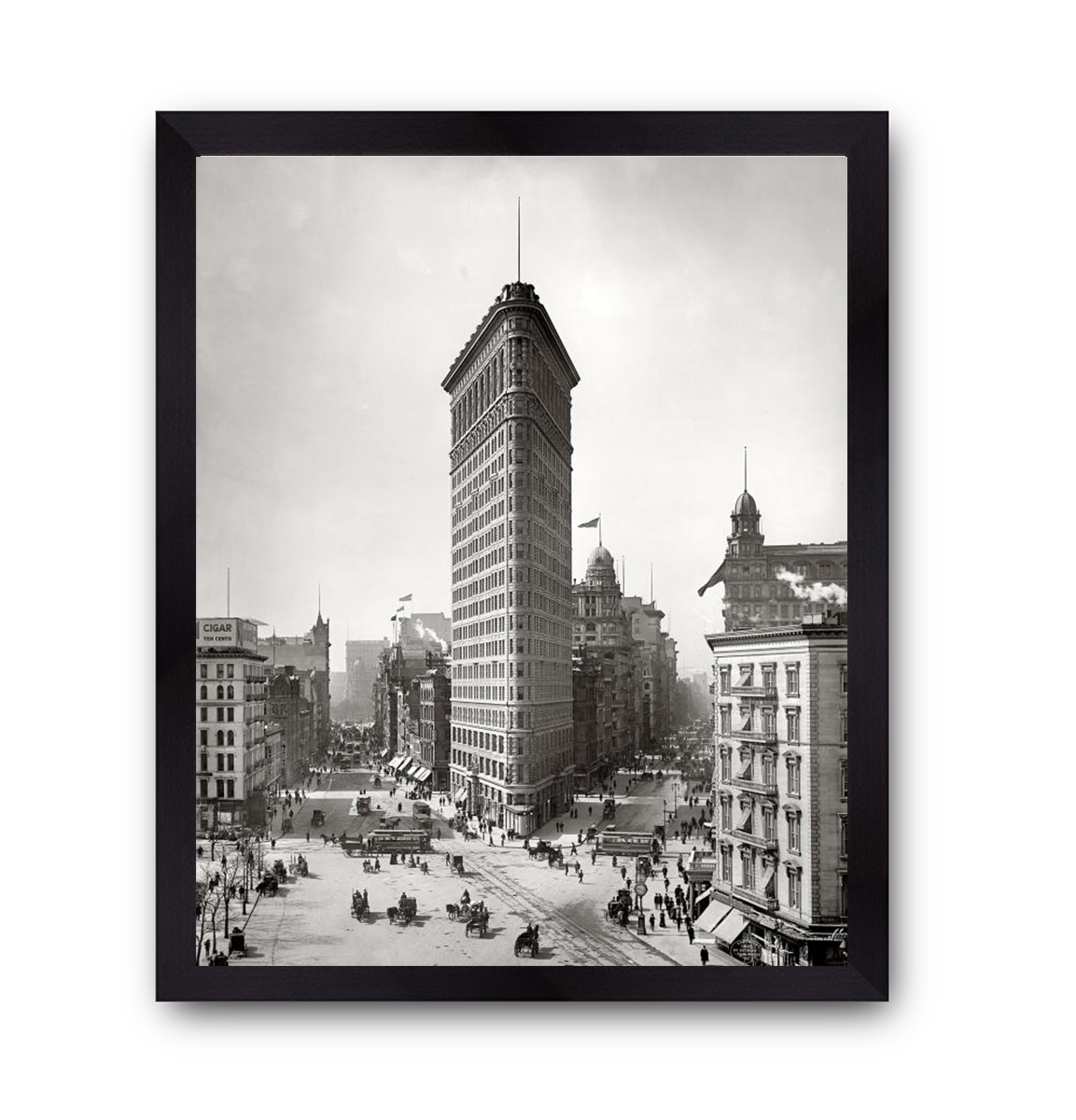The image appears to be a black-and-white photograph taken around the turn of the 20th century, capturing a historic view of New York City. Central to the composition is the iconic Flatiron Building, a triangular-shaped structure standing between 20 to 30 stories tall, positioned where the streets diverge to the right and left. This prominent feature faces the viewer with its pointed front, showcasing early 20th-century architecture. Surrounding the Flatiron Building are smaller, low-rise buildings, with a notable large building in the right corner adorned with awnings. The streets are abuzz with activity, filled with people walking the sidewalks and horse-drawn carriages traversing the roads, alongside some early buses, highlighting the era's transportation. Streetlights illuminate the pathways, barren trees punctuate the scene, and flags wave atop several buildings, including a tower visible in the right background. The sky is a bright shade of white, further emphasizing the vintage charm of this early New York City tableau.